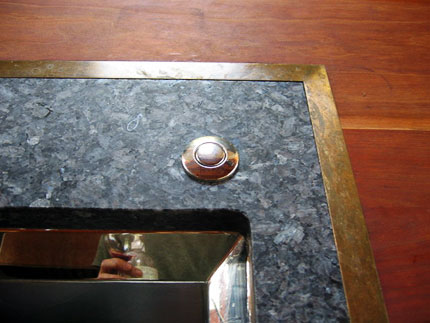The image depicts a section of a wooden structure with intricate details. Starting from the top left, a wooden panel extends down approximately two inches and then extends horizontally to the right, stopping two inches from the edge. From this point, the wood slopes downward at an angle towards the right. The upper section and the right side of the image are dominated by rich brown wood.

Within this wooden frame, there's a gold border that runs down towards the left. About an inch below where this gold border intersects, there is a small striation in the wood resembling a divot. Moving inward from the gold border, a marble-like floor surface emerges, extending about two inches downwards on the left side and approximately an inch on the right side.

Positioned near the bend where the gold border angles, there is a circular feature with a gold outline, containing what appears to be a push button. Below this, the marble surface transitions into what seems like a mirror, reflecting a glimpse of the brown wood flooring.

Beneath the button, a person wearing a green shirt is visible. Additionally, there is a clear soap dispenser with a white top, and on its left side, a hand with the pointer finger wrapped around the dispenser can be seen. At the very bottom of the frame, a thin silver piece extends from the left, runs horizontally almost to the opposite border, and then descends.